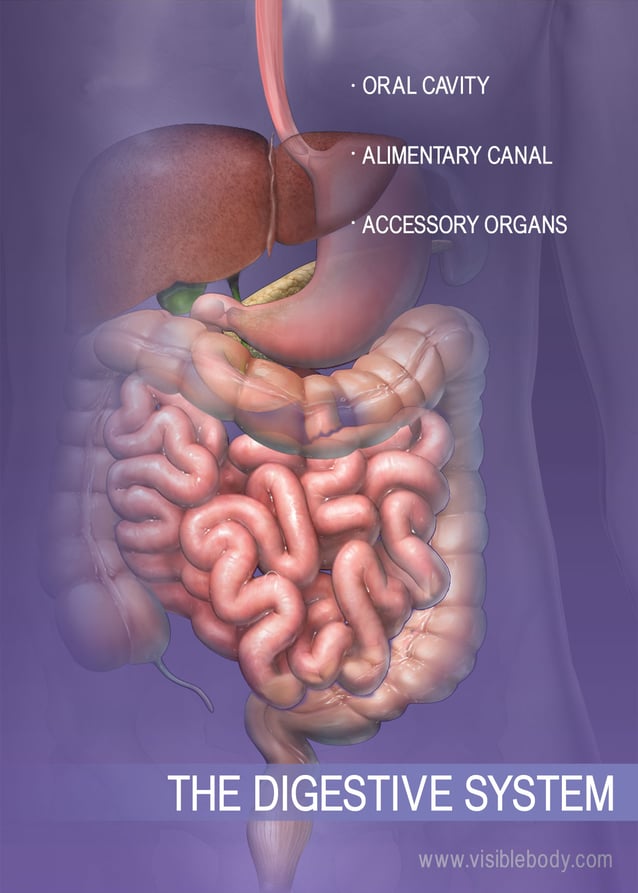Displayed is a detailed and colorful computer-generated illustration of the human digestive system. The image, predominantly in shades of medium and lighter purple, features the label "The Digestive System" and the URL "www.visiblebody.com" emblazoned in white across the bottom stripe. 

The diagram spans from the esophagus to the colon, showcasing all intermediary organs. The subject headings to the right of the image are "Oral Cavity," "Alimentary Canal," and "Accessory Organs." The background contains a faint outline of the human body in blue-gray hues, enhancing the focus on the digestive tract itself, which is vividly depicted in an array of colors from pink to reddish-brown.

Visible components include the oral cavity, the stomach prominently positioned above the intestines, and the small and large intestines. Details down to the tiny appendix at the lower part of the large intestine are seen, illustrating their placement as they naturally occur. The image provides a comprehensive and educational view of the digestive system, highlighting essential organs like the liver and the excretory pathways within the context of the human anatomy.